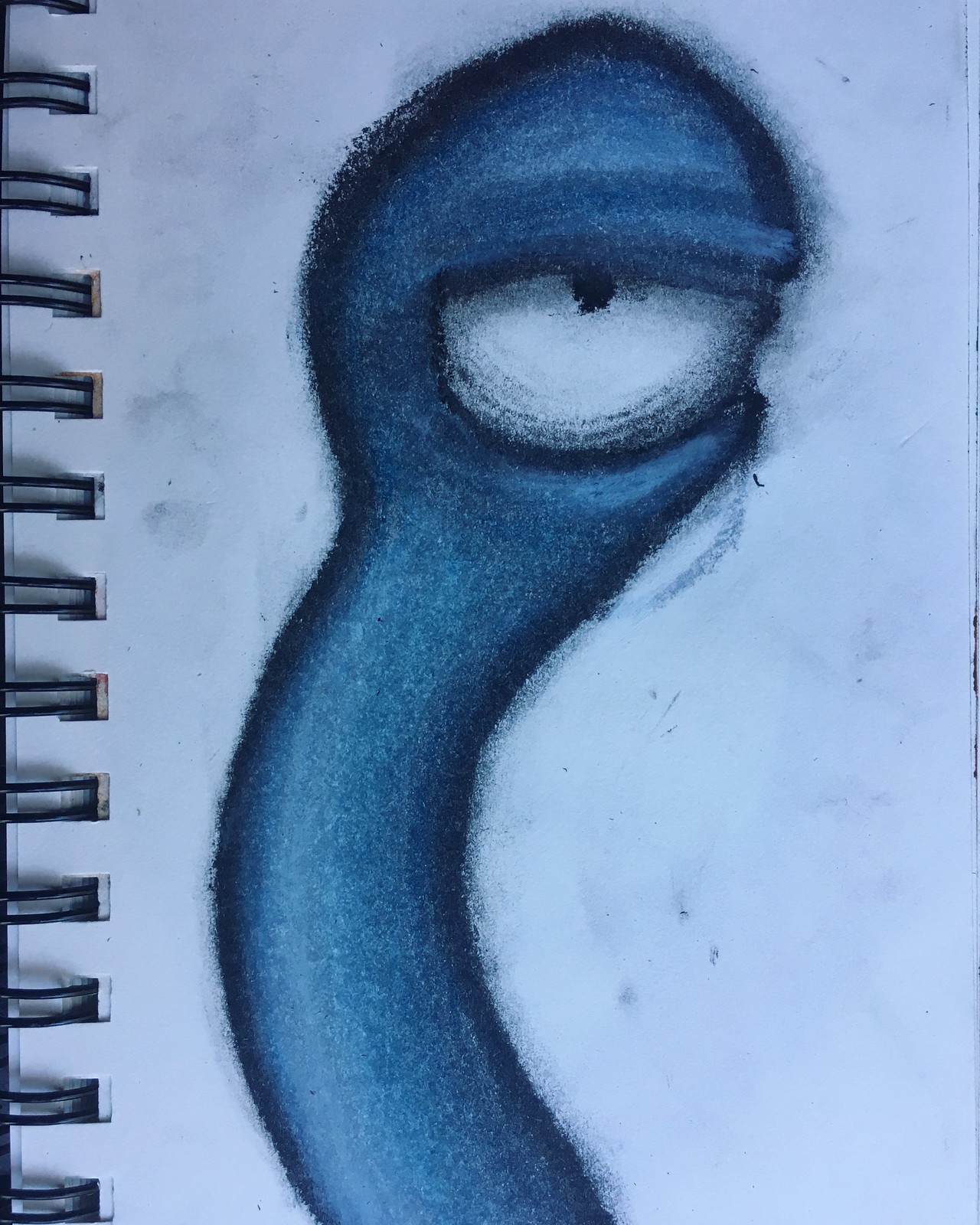In this drawing found in a sketchbook, the illustration is set against white paper marred with stains in various darker hues such as blacks, grays, and dark blues. On the left side of the image, the notebook's binding is visible, anchoring the composition. Executed in a scratchy, rough medium, the artwork depicts a peculiar creature characterized by a single, prominent eye perched on a lengthy, neck-like stalk. The stalk gracefully curves slightly to the left before bending back over, culminating in a round head. The creature's solitary eye is half-lidded, exuding a weary expression, with the pupil directed upward in a tired gaze. The shading in this piece employs a spectrum of colors; light caresses the left side of the creature's neck and its head, while deeper shadows envelop the right side and the underside of the eye.